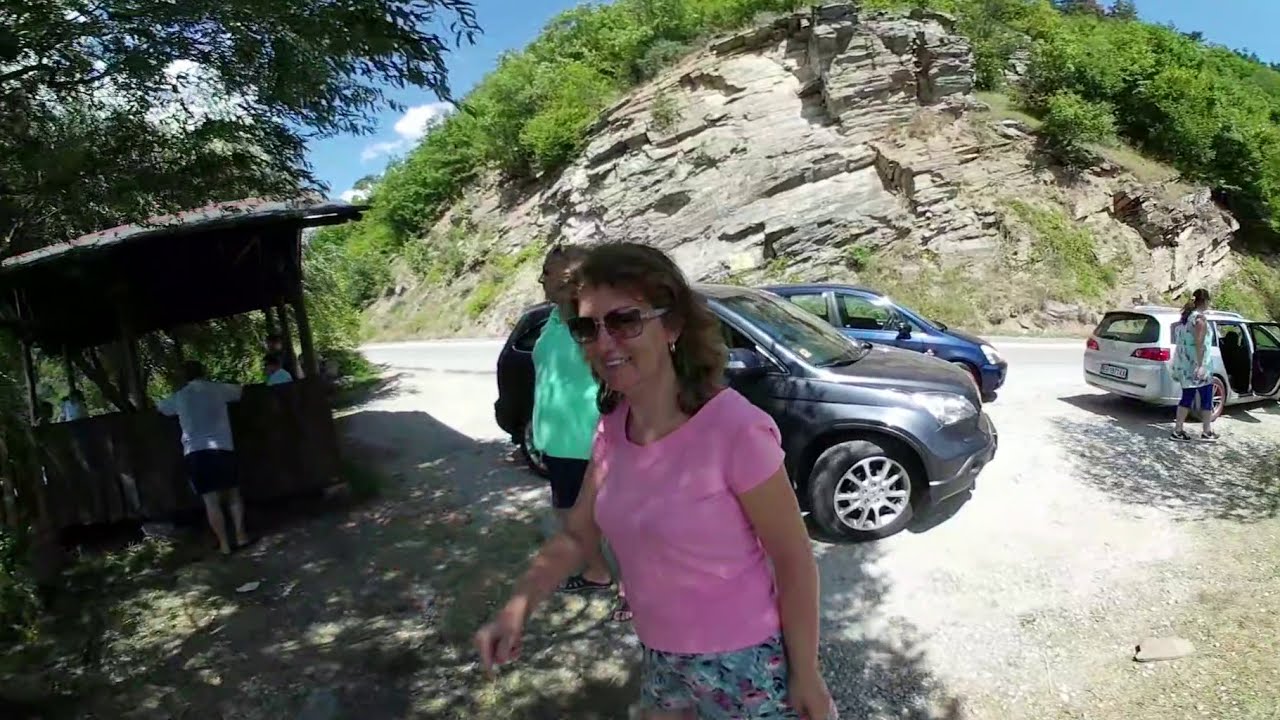In the photograph taken on a bright day, a woman with curly brown hair, wearing sunglasses, a pink shirt, and blue floral print shorts stands prominently in the foreground. Behind her is a man in a teal shirt and black shorts. To the left, a wooden gazebo with a thatched roof shelters a few people seated inside, while a person in a white shirt leans into it. A grey SUV is parked behind the man, with a blue minivan and a white car further to the right. A woman in teal capri pants and a light blue tank top is walking towards the right side of the image. In the background, a large rocky hill covered with green bushes and grass looms over the scene, adding natural beauty to the vivid and diverse colors of the composition. The overall setting is well-lit by natural daylight, emphasizing the vibrant atmosphere of the outdoor location, which appears to be a scenic area beside a road, possibly a canyon or some form of natural park.